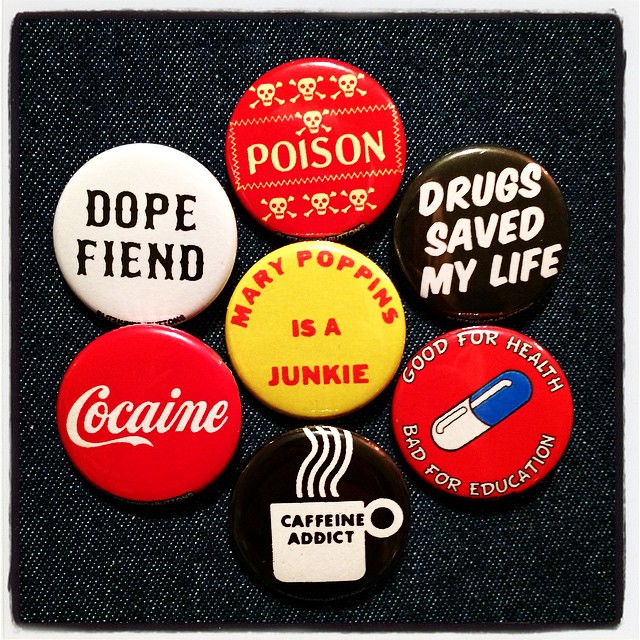The image displays an array of seven metal buttons pinned to a piece of dark denim, possibly black or dark blue. These buttons, often used as accessories for clothing, feature distinct designs and messages:

- At the top center, a red button with white text reads "POISON" and is adorned with multiple skull faces.
- Directly to the left, a white button with black text displays the phrase "DOPE FIEND."
- Just beneath these, a yellow button with red text states "Mary Poppins is a junkie."
- Below the "Dope Fiend" button, a black button with white text proclaims "DRUGS SAVED MY LIFE."
- Positioned underneath is a red button bearing the phrase "Good for health, bad for education" in white text, split by a blue and white pill graphic.
- At the bottom, a black button features a white coffee mug with spirals of steam and the text "CAFFEINE ADDICT."
- To the right, a red button replicates the Coca-Cola logo but with the word "COCAINE."

Each of these buttons shares a theme relating to substances and addiction, contributing to a cohesive yet provocative message.